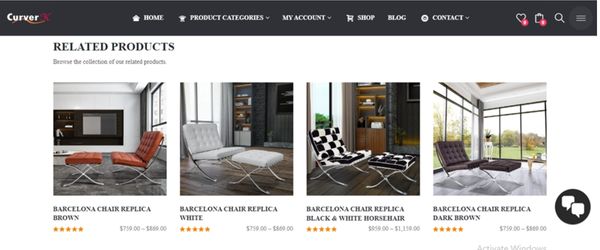The webpage showcases various chair products under the brand "Curver," whose logo is displayed at the top left corner. The black banner across the top features navigation tabs for Home, Product Categories, My Account, Shop, Blog, and Contact, accompanied by icons for favorites (heart), messages, and search.

The center of the image prominently displays a collection of chair photographs labeled as related products. The first chair is a red Barcelona Chair replica with a distinctive split backrest, priced with a five-star rating. Next, a white Barcelona Chair replica is situated in an indoor setting with a window and visible flooring, also rated five stars. Following this is a checkered black and white horsehair Barcelona Chair replica, again boasting a five-star rating.

The last chair in the collection is a dark brown Barcelona Chair replica, designed to accommodate two people with an accompanying footrest split in the center. The price details reveal the horsehair version starts at $959, while both the white and brown Barcelona Chair replicas are priced starting at $759.